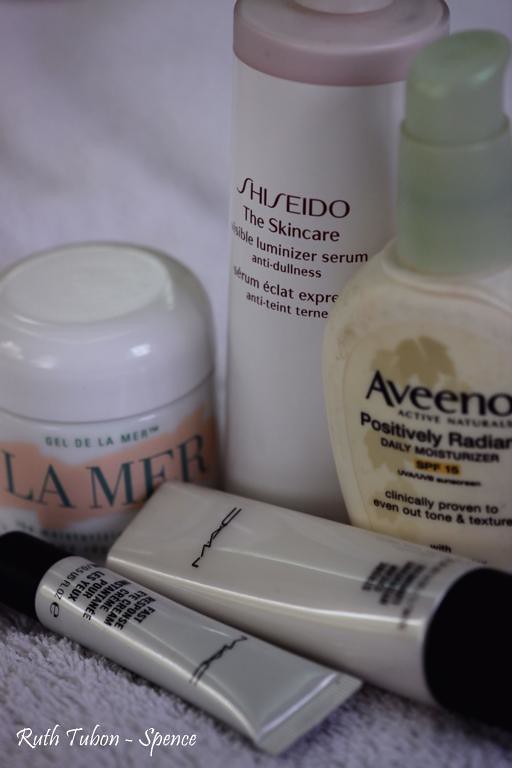A meticulously organized skincare collection is showcased in this image, set against a light gray background that could either be a towel or carpet, adding a soft texture to the scene. The bottom left corner features a watermark in italic white font reading "Ruth Tubon-Spence."

At the heart of the collection is a Shiseido Visible Luminizer Serum promising anti-dullness benefits. To its immediate right stands an Aveeno Active Naturals Positively Radiant Daily Moisturizer with SPF 15, boasting UVA and UVB protection and claims of clinically proven effectiveness for even skin tone and texture. Below the Aveeno moisturizer are two MAC products: one appears to be a primer, though the exact labeling is blurred, and the other is a small tube of MAC Fast Response Eye Cream.

Positioned above the MAC products and to the left of the Shiseido serum is a luxurious jar of La Mer cream in its iconic white packaging. Adding a touch of contrast, a white piece of fabric subtly peeks from the background, enhancing the overall aesthetic of the display, which balances utility and elegance.